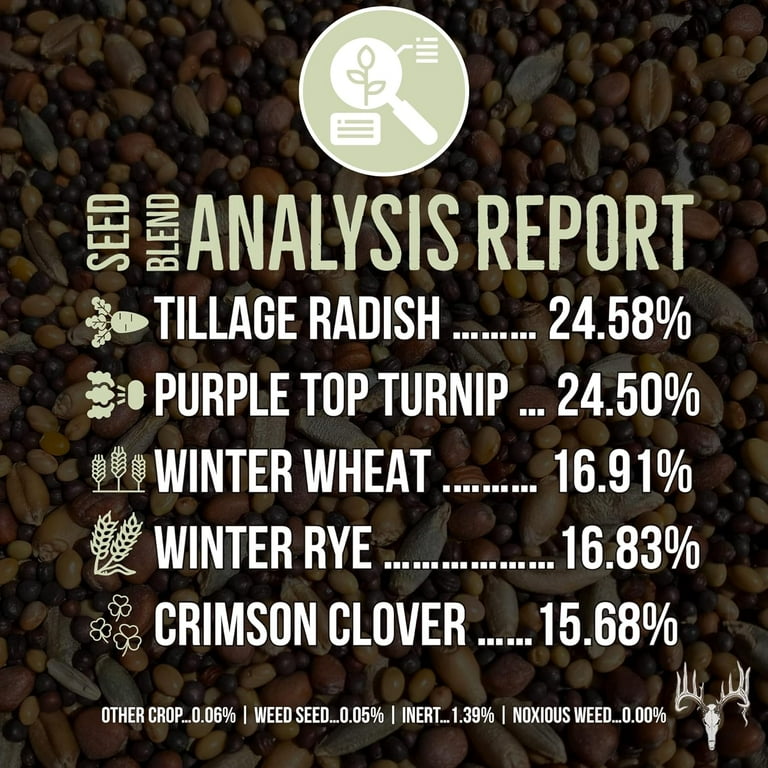The image is a square-shaped, six-inch by six-inch seed blend analysis report, set against a slightly darkened background of various seeds, grains, and beans of different shapes, sizes, and colors. The focus is on the text overlay. At the top center, there is a green circle with a white outline, featuring an icon of a magnifying glass with a plant symbol inside. The text "Seed Blend" is printed vertically in green, with "Analysis Report" written horizontally to the right in white letters. 

Below the title are five rows depicting different seeds, each row having a green illustration of the seed on the left and the corresponding name and percentage on the right in white text: Tillage Radish (24.58%), Purple Top Turnip (24.50%), Winter Wheat (16.91%), Winter Rye (16.83%), and Crimson Clover (15.68%). At the bottom, smaller white print details the minor components: Other Crop (0.06%), Weed Seed (0.05%), Inert Matter (1.39%), and Noxious Weed (0.00%). In the lower right corner, there is a white stamp of a deer skull with antlers.